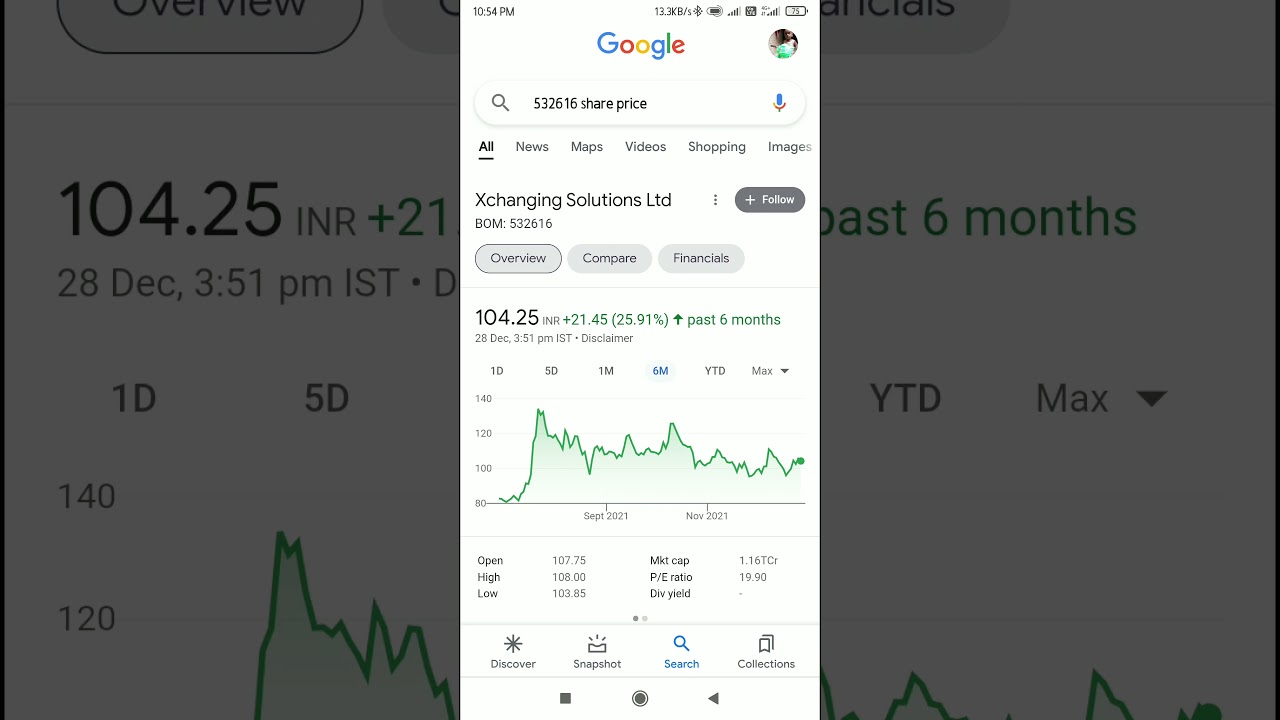The image captures a screenshot of a Google search conducted on a smartphone, as indicated by the narrow screen dimensions and the display of phone-specific icons, such as battery life and the time shown as 10:54 p.m. The interface exhibits Google's iconic logo in blue, red, gold, and green colors. The user has searched for "532616 share price," and the Google search bar is accompanied by the Google microphone symbol. The search results feature a highlighted "All" tab and present data related to a company named "Exchanging Solutions Limited."

Prominently displayed is the company's stock price, $104.25, which has risen by $21.45, marking a 25.91% increase over the past six months. Below the stock price, a graph is shown with a jagged dark green line overlaid on a light green background, illustrating the stock's movement from September 2021 to November 2021, where the price starts to increase and then steadies. Information about the stock includes opening, high, low prices, market cap, PE ratio, but no data for the dividend. At the bottom of the screen are app icons characteristic of a smartphone interface, suggesting navigation options. The entire screenshot appears layered over another, slightly obscured webpage, giving a grayish, faded backdrop effect.